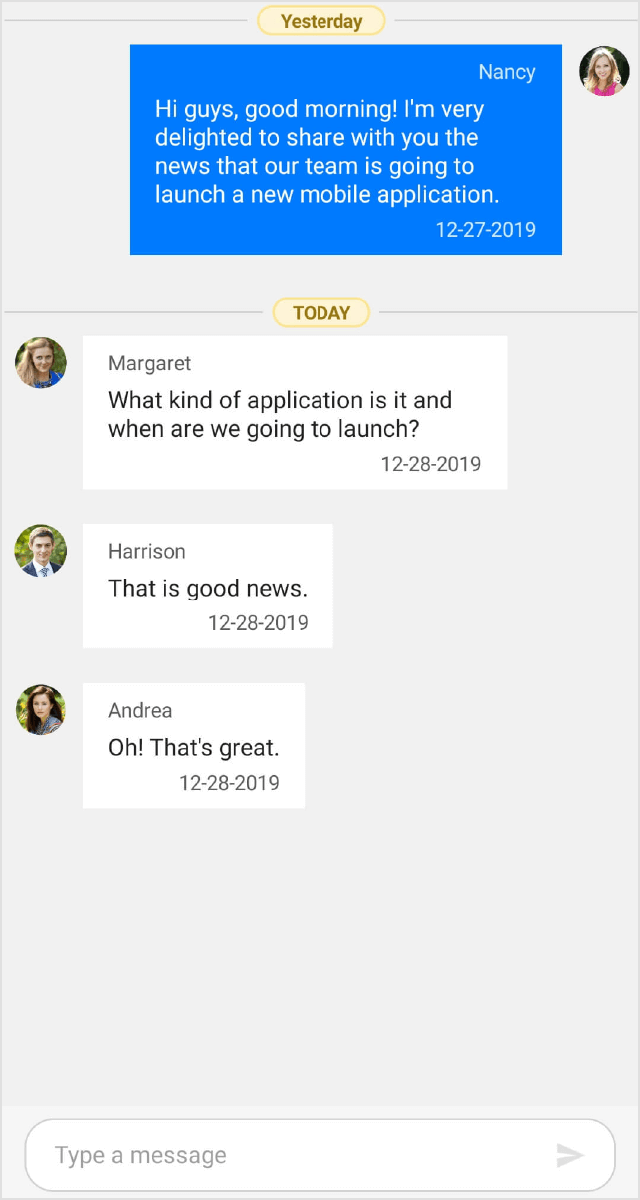The image features a gray background with a yellow oblong-shaped box at the top, displaying the word "Yesterday" with light gray vertical lines on either side. Below this, in a vibrant blue box, is the message: "Hi guys, good morning. I'm very delighted to share with you the news that our team is going to launch a new mobile application." It is signed "From Nancy on December 27, 2019," accompanied by a small profile picture that appears to depict a person with blonde hair.

Further down, there is another yellow oblong-shaped box with the word "Today" and similar gray vertical lines on either side. Below this, a white box contains a message from Margaret: "What kind of application is it and when are we going to launch?" dated December 28, 2019. Beneath Margaret's message, Harrison comments: "That is good news," also dated December 28, 2019. Following Harrison's comment, Andrea expresses her excitement, saying: "Oh, that's great," with the date noted as 12-28-2019.

At the very bottom of the image, there is a text box, suggesting an input area for further messages or comments.